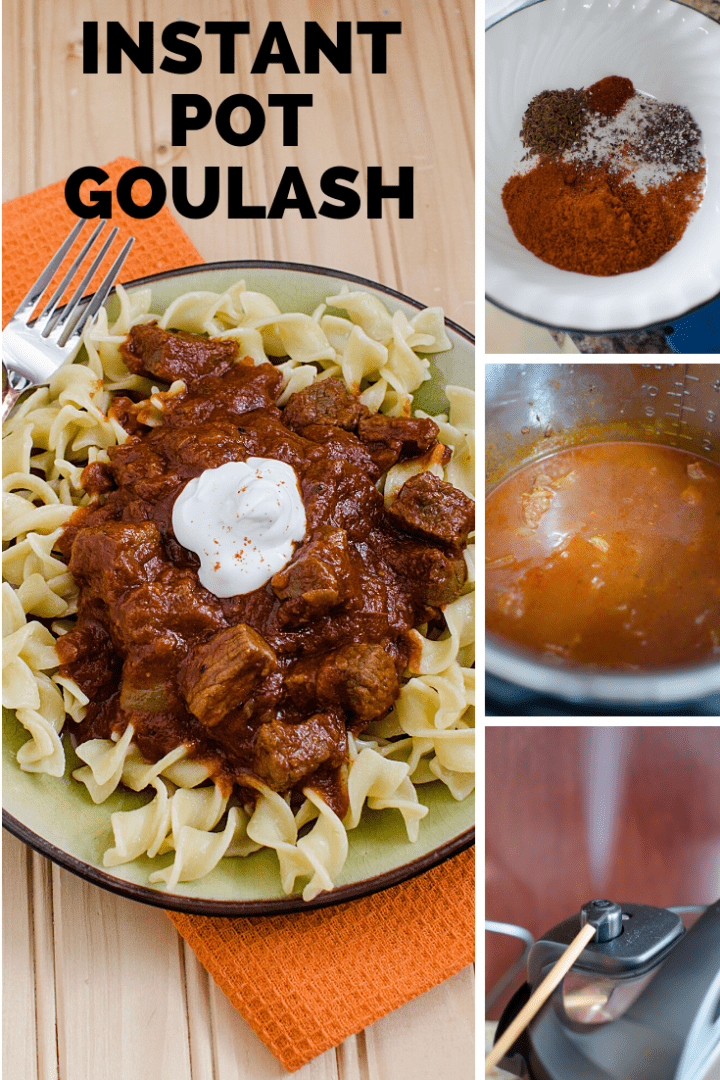The image is a detailed collage consisting of four photographs arranged with one large image on the left and three smaller images stacked vertically on the right. The prominent left photograph showcases a plate labeled "Instant Pot Goulash" in black text at the top. The dish features elbow pasta in a thick yellow hue, bathed in a dark red sauce, and finished with a dollop of white sour cream in the center. Accompanying the plate is a silver fork positioned towards the top left, resting on a thick light green napkin. The light green plate with black edges sits atop a light brown wooden table.

Moving to the right side of the collage, the topmost image depicts a white bowl filled with a blend of dry ingredients or spices, displaying colors such as orange, white, and dark brown. The central image offers a close-up view of the cooking process within a silver, metallic pot, containing an orange or reddish-brown soup-like mixture. Finally, the bottom image focuses on a part of an object that resembles a manual can opener or cooking device, with a thin yellow strand or stick next to it, and steam emitting from the black Instant Pot lid. The entire collage is bordered with small white lines separating each photograph.